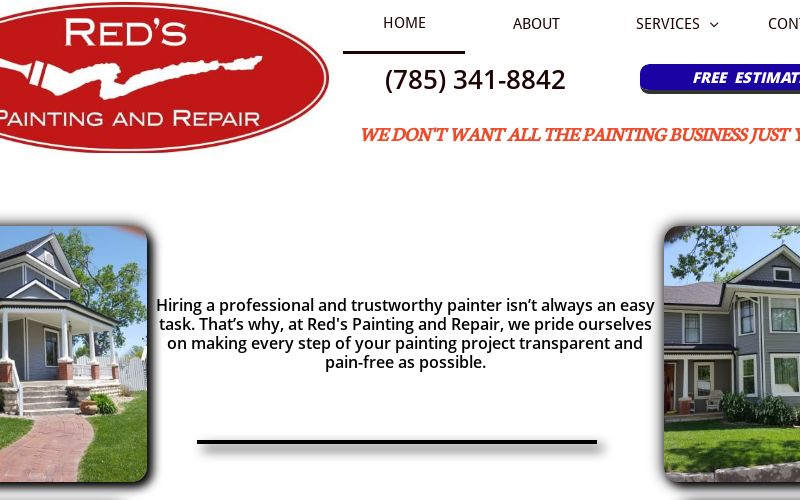In the top left corner of the image, there is a prominent red oval logo with a slender white border, followed by a thin red border. Inside this oval, "RED'S" is displayed in bold, capitalized white letters. Adjacent to the text is a white icon of a paintbrush, which appears to be painting a streak of white paint. Below the logo and slightly cut off on the left, about one-fifth, the text "PAINTING AND REPAIR" is written in smaller, capitalized white letters.

To the right of the logo, there is a navigation menu listing "HOME," "ABOUT," "SERVICES," and partially visible "CON..". "HOME" is underlined with a thick black line, indicating it is currently selected. Next to "SERVICES," a downward arrowhead suggests the presence of a dropdown menu. Directly beneath the menu, a phone number, "(785) 341-8842," is displayed in bold black font.

Next to the phone number is a blue, slightly 3D button with rounded corners labeled "FREE ESTIMATES," though the text is cut off at the "T." Below this, an orange italicized font reads, "we don't want all the painting business just," but it appears to be cut off at the completion of the word, presumably transitioning to "yet."

Towards the bottom left of the image, there is a picture of a gray house with a well-maintained lawn and a brick walkway. Centrally positioned in black font, a testimonial reads: "Hiring a professional and trustworthy painter isn't always an easy task. That's why at RED'S PAINTING AND REPAIR, we pride ourselves on making every step of your painting project transparent and as pain-free as possible."